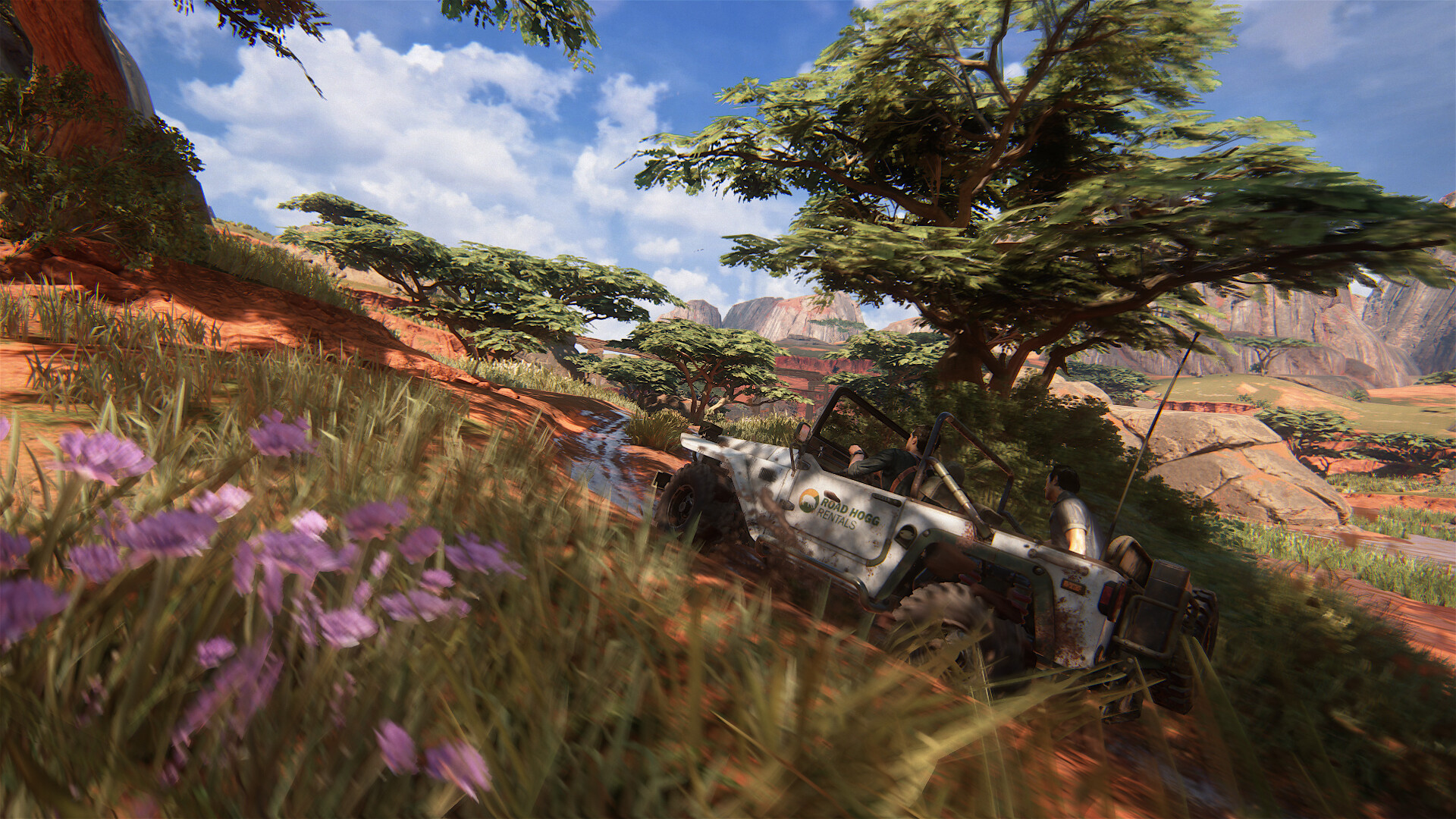This image is a highly detailed screenshot from a video game, most likely from the Uncharted series. It showcases a rugged, desert-like environment with a distinct red clay ground and small, flat-topped green trees that resemble those found in African or Australian landscapes. Central to the image is a white, convertible jeep-style vehicle labeled "Roadhog Rentals," driven by two Caucasian men with dark brown hair. One of the men, who appears to be Nathan Drake, the protagonist from the Uncharted series, is dressed in a dark gray shirt. The other passenger wears a green jacket. The vehicle, equipped with rugged tires, navigates an uphill dirt trail dotted with wet ruts. The foreground features patches of grass sprouting light purple flowers, adding a splash of color. In the background, large rock formations and boulders punctuate the bright blue sky adorned with several puffy white clouds, completing this picturesque and adventurous scene.